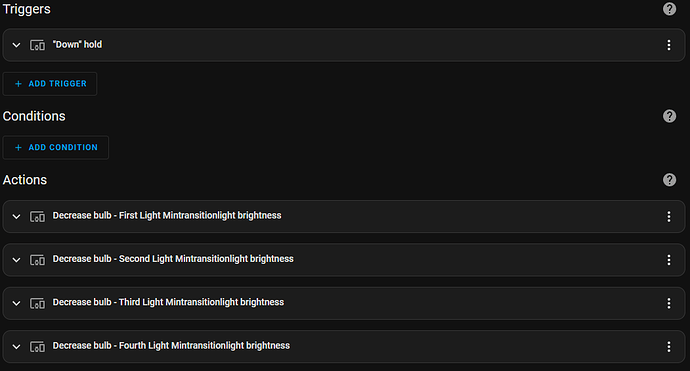The image captures a screenshot of a computer interface displaying settings for trigger-based automation. At the top, there is a highlighted section labeled "Triggers," beneath which is an entry titled "Down (Hold)." This entry includes icons of a computer and a cell phone beside it, indicating it is a multi-device trigger. To the far right of this entry, three dots suggest additional options or information can be accessed.

Below this, there's a section titled "Blueprint," with a rectangular button labeled "+ Add Trigger." Following that, a section named "Conditions" appears, also featuring a rectangular button labeled "+ Add Condition." Both rows have a question mark at the end, hinting at help or more information available.

Next, there's an "Actions" section, marked similarly with a question mark at the end of the row. This section contains four entries, each designated with a downward-pointing arrow and labeled as follows:
1. “Decrease Bulb First Light Mini-transition Light Brightness”
2. “Decrease Bulb Second Light Mini-transition Light Brightness”
3. “Decrease Bulb Third Light Mini-transition Light Brightness”
4. “Decrease Bulb Fourth Light Mini-transition Light Brightness”

Each entry is formatted within a rectangular box, indicating that they are part of a sequence of actions to be carried out.